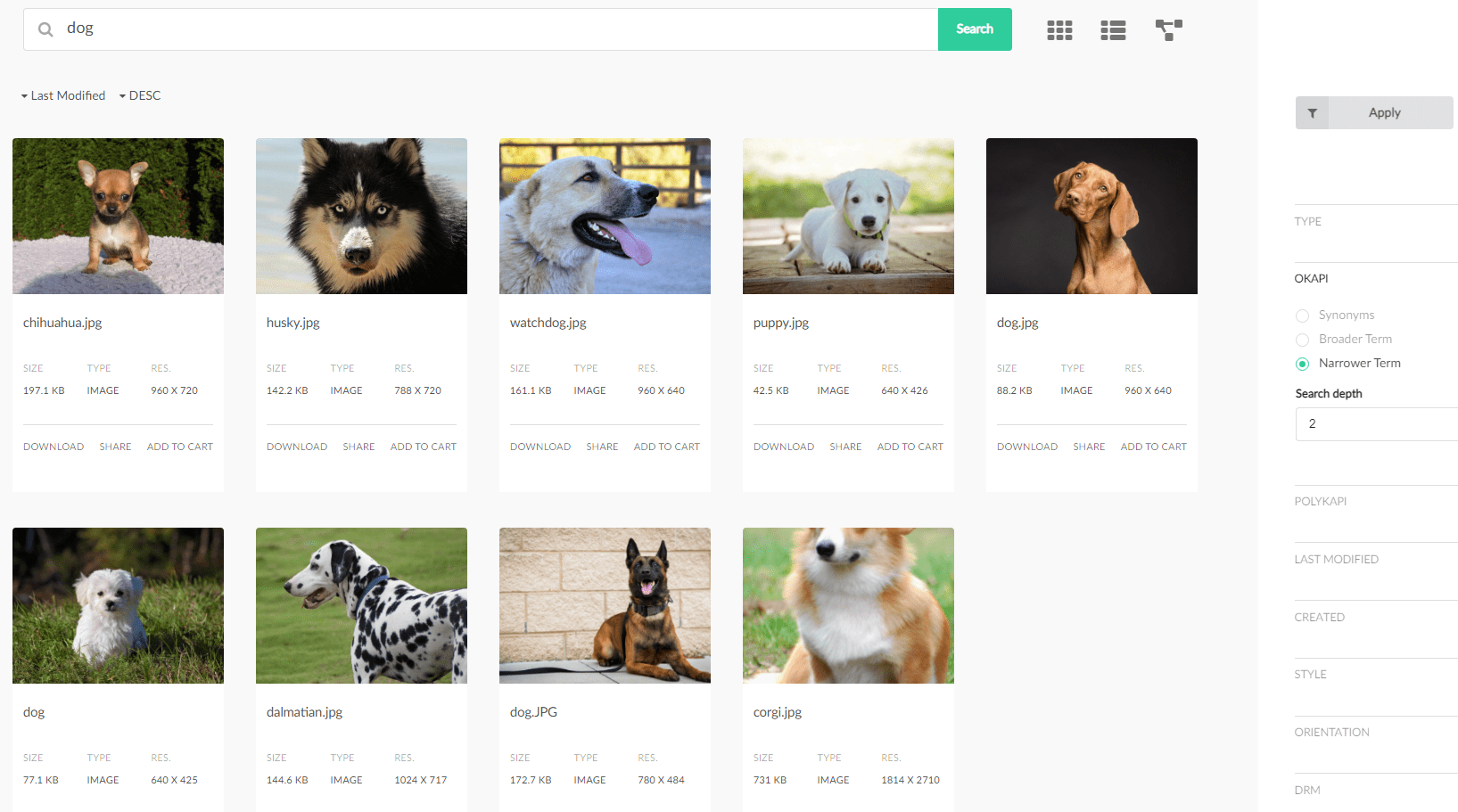A collection of various dog pictures is displayed, all tagged in a search bar under the keyword "dog" with unspecified modification dates and limited descriptions. The images feature:

1. A cute little brown Chihuahua, showcasing its tiny stature and big, expressive eyes.
2. A striking Husky with its signature thick fur and piercing blue eyes.
3. A vigilant Watchdog, exuding alertness and strength.
4. An adorable puppy, embodying the essence of youthful playfulness and innocence.
5. A unique mixed breed that resembles a bloodhound, with a shiny coat and a distinctive look.
6. A fluffy little white dog, exuding charm with its soft, cloud-like fur.
7. A Dalmatian, displaying its iconic black spots on a sleek, white coat.
8. A German Shepherd, marked simply as "dog," with a brown and black coat and a notably black face.
9. A Corgi, whose photo is partially cropped just above its eyes, leaving the viewer to imagine its complete, expressive face.

All filenames follow the pattern "type of dog.jpg," adding a layer of uniformity to the collection.